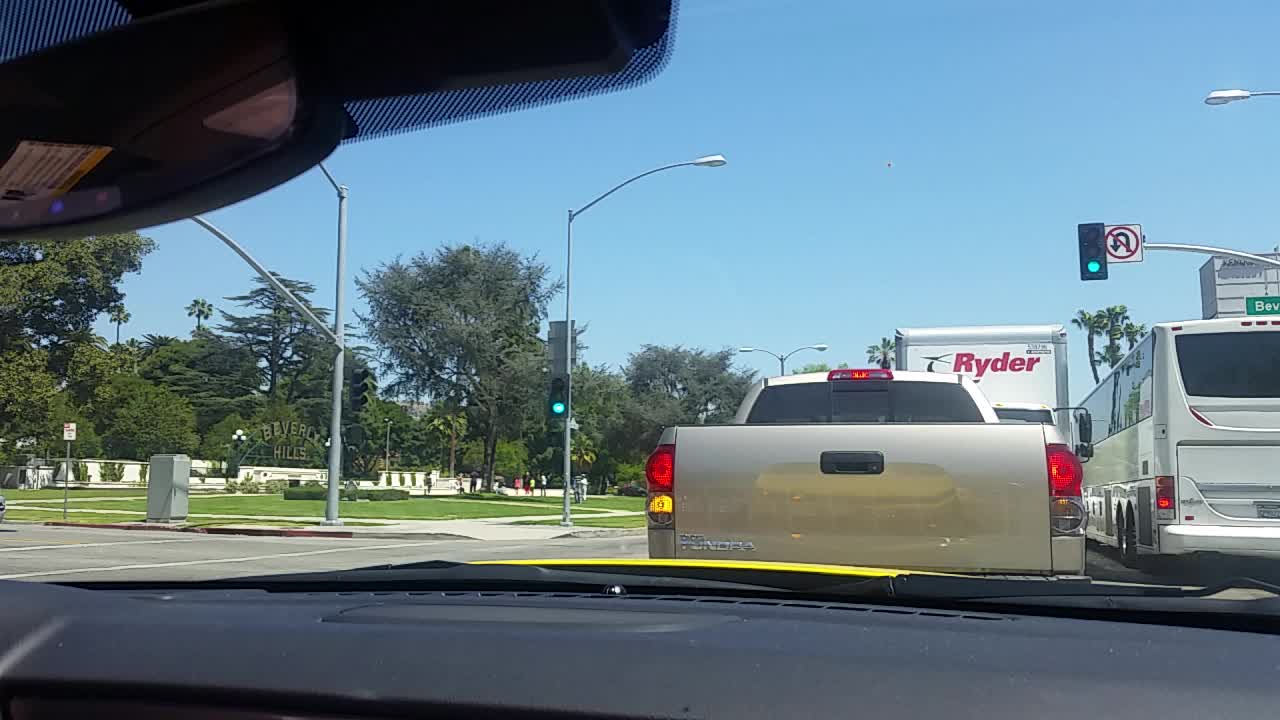Under a bright blue sky, this photograph captures a vivid outdoor scene viewed from inside a car. To the left, a grassy area leads up to a line of trees in the background. Two tall light poles stand at the corner of a cement sidewalk, each curving gracefully upwards. Visible through the car's rear-view mirror, the dashboard provides context hinting at the driver's perspective. To the right, a green traffic light is visible, accompanied by a street sign signaling that U-turns are prohibited, marked with a curved arrow inside a circle with a slash. Further ahead, there is a large white bus and an imposing truck bearing the name "Ryder" spelled out in bold letters. The juxtaposition of natural elements and urban utilities, coupled with the in-car viewpoint, adds layers of depth to the scene.